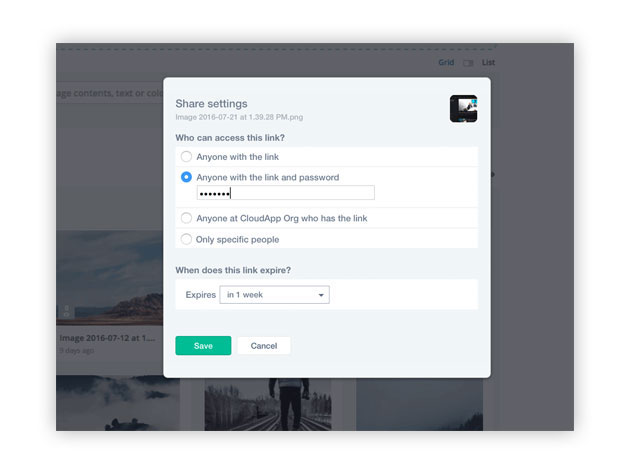The image displays a user interface with a light blue background, focused on sharing settings for a specific image file. At the top of the interface, there's a darker blue header that reads "Share Settings." Below this header, the image filename "image 2016-07-21 at 1.39.28pm.png" is displayed. The section below inquires "Who can access this link?" with selectable options in a white box. 

There are multiple radio button options, which turn blue when selected. The options include: 
1. "Anyone with this link"
2. "Anyone with the link and password" (this option is selected, and a password is entered, revealed by the presence of obscured dots)
3. "Anyone at the cloud app or who has the link"
4. "Only specific people"

Further down, there's a section asking, "When does this link expire?" with another white box stating "Expires in one week." At the bottom, two rectangular buttons are displayed: a green and white button labeled "Save" and a grey and white button labeled "Cancel."

In the shaded gray background behind this interface, there's a faint, partially obscured image of a person walking on train tracks. On the left-hand side of the interface, beneath the sharing options, there's some barely readable text: "image 2016-07-12 at 1.... golden cross."